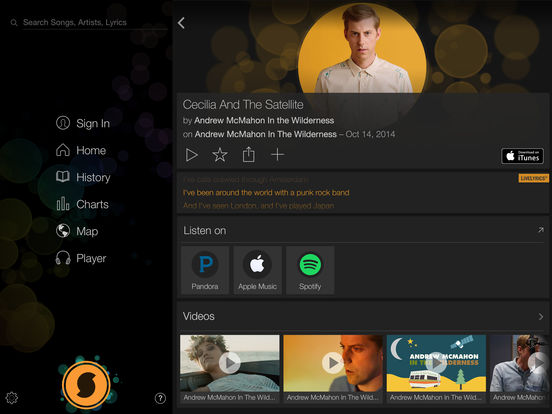A screenshot of a music player app, prominently displaying a search bar on the left with options to search for songs, artists, or lyrics. The interface includes navigation tabs such as 'Sign In,' 'Home,' 'History,' 'Charts,' 'Map,' and 'Player.' The currently selected song is "Cecilia and the Satellite" by Andrew McMahon in the Wilderness, released on October 14th, 2014. The song's artwork features a person with a yellow background, serving as Andrew McMahon's avatar. The app suggests listening to the track on platforms like Pandora, Apple Music, or Spotify. At the bottom of the screen, additional videos by Andrew McMahon are listed, indicating this is his dedicated channel, highlighted by the quote: "I've been around the world with a punk rock band."